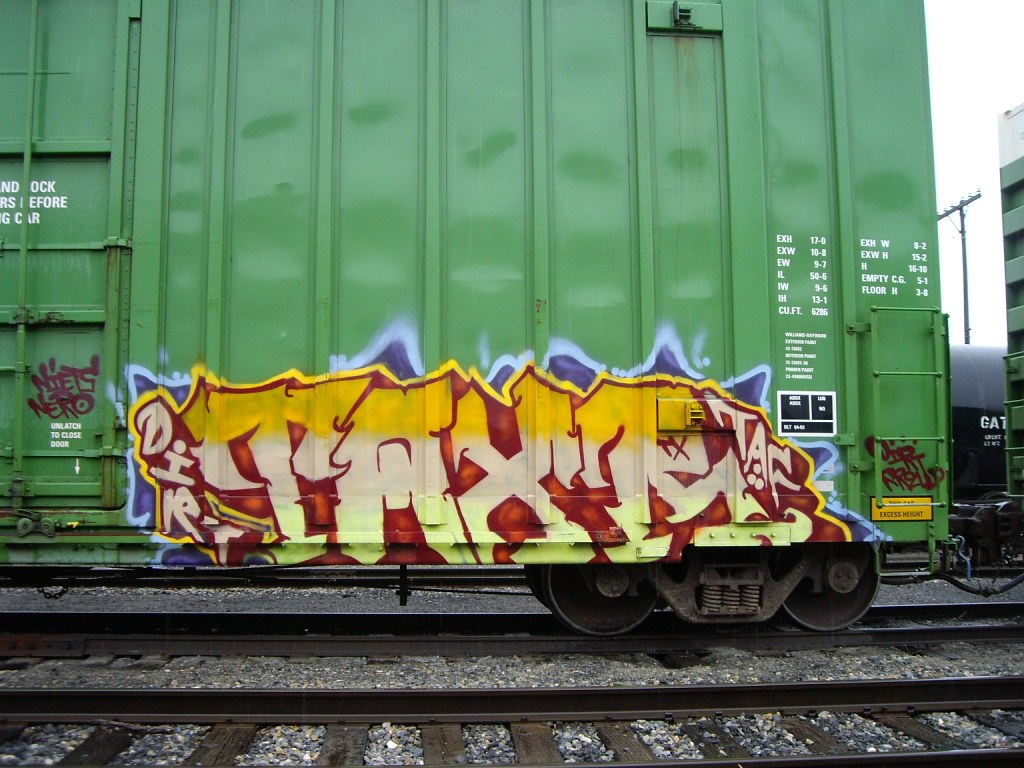The photograph captures a meticulously maintained, green-painted, corrugated steel train car, seemingly new and positioned on a well-kept railway track in a train yard or station. The train car features sturdy vertical support bars, a lock doorbar on the left, and a visible small ladder on the bottom right. There is white informational lettering on the metal body of the car. 

Prominently, the lower half of the door displays a complex layer of graffiti. Dominantly present is a stylized tag featuring yellow and white gradient letters spelling out "TAXF" or similar, intersected vertically by "DIHR." This new graffiti partially obscures an older blue one beneath it. Flanking this main artwork, smaller tags include a maroon piece on the left reading "Nietz Nero" and another burgundy tag under the ladder on the right with partially legible text, possibly saying "Dirt Around, Dirt Proud." Alongside the train car, the railroad track is visible with its brown rails and gravel base, indicating a clean and functional infrastructure.